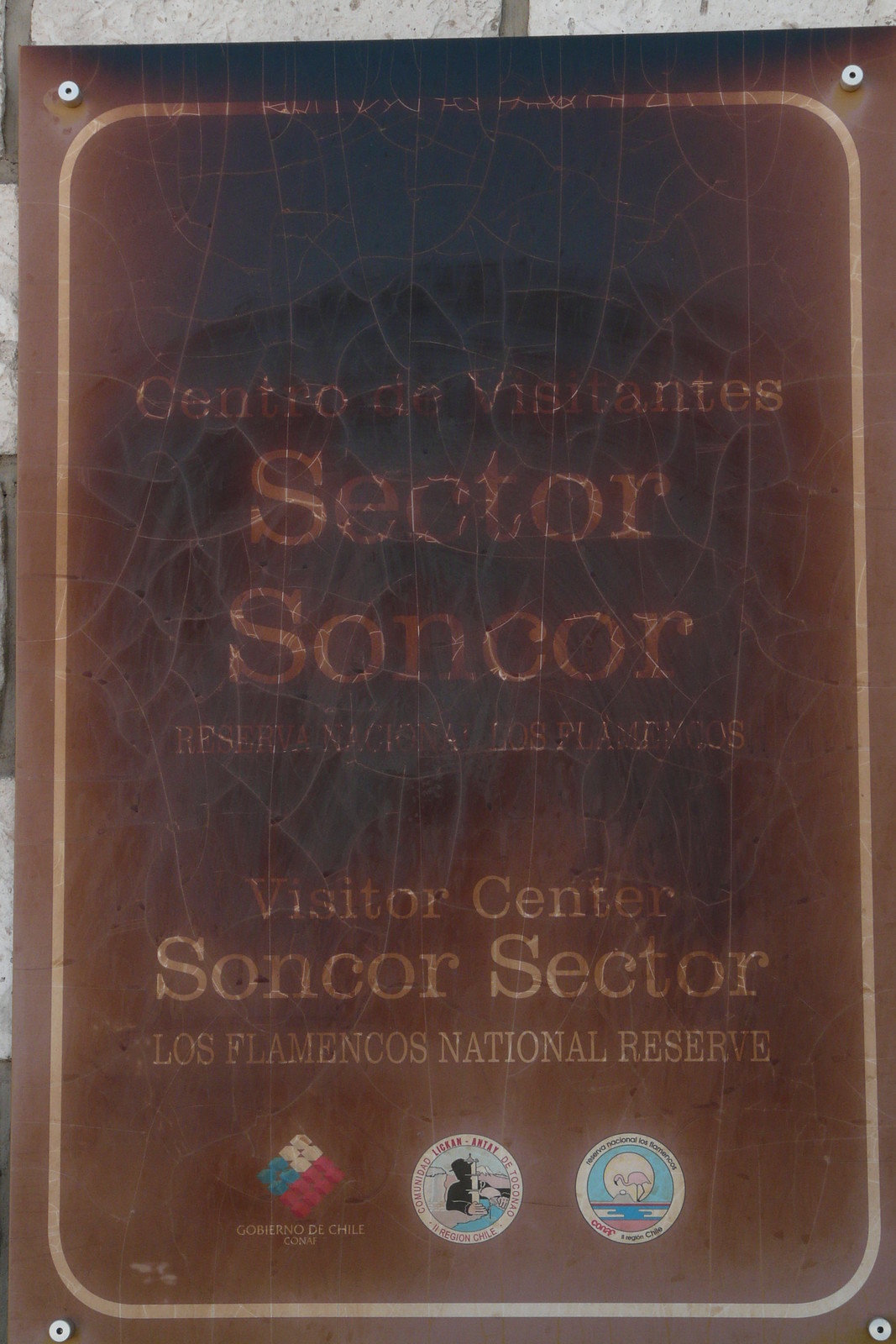This image captures a close-up of a heavily weathered plaque secured to a white brick or stone wall using four brass rivets at each corner. The plaque is predominantly dark brown, almost appearing black due to extensive sun damage and wear, giving it a faded and discolored look. Despite the wear, some of the text is discernible. The top of the plaque displays text in Spanish, which includes "Centro de Visitantes" and "Sector Sancor." Directly below, in slightly larger and still legible white letters, it reads "Visitor Center, Sancor Sector, Los Flamencos National Reserve." The lower portion of the plaque features three logos: the first on the left is red, white, and blue in the shape of a diamond, marked with "de Chile" beneath it. The other two logos are circular, containing words and symbols that are largely indecipherable due to the plaque's extensive weathering and accumulation of grime. The plaque's beveled edges are also noted to have a beige border that has succumbed to the elements, adding to its aged and dirty appearance.